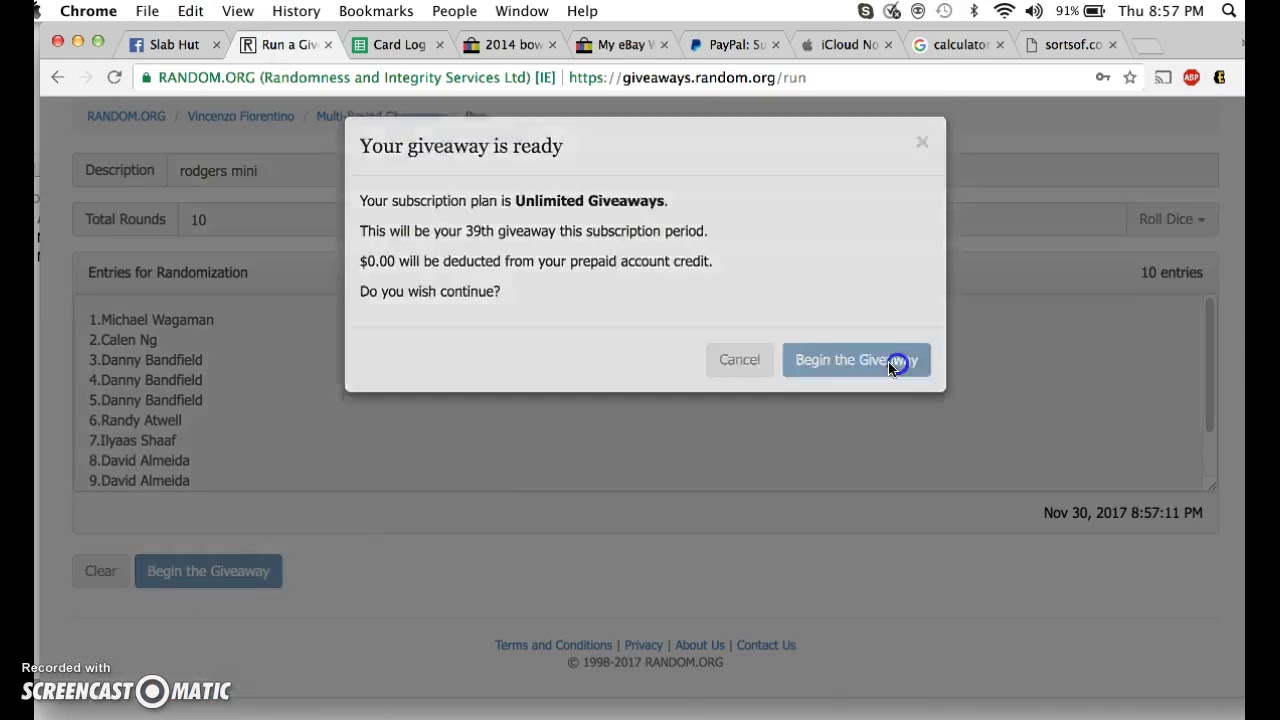**Detailed Caption:**

The image depicts a web page open on Google Chrome with a total of nine tabs visible at the top. The currently active tab is displaying a page from random.org, specifically "http://giveaways.random.org/run." Dominating the center of the screen is a pop-up box, partially obscured by a gray overlay over the rest of the web page. The pop-up box contains the following text, which is prominently highlighted:

**"Your giveaway is ready. Your subscription plan is UNLIMITED GIVEAWAYS"** (with "UNLIMITED GIVEAWAYS" in bold).

The message continues: 

**"This will be your 39th giveaway this subscription period. $0 will be deducted from your prepaid account credit. If you wish to continue, please click 'Begin the giveaway'."**

At the bottom of the pop-up, there are two buttons: "Cancel" and "Begin the giveaway." The cursor is seen hovering over the "Begin the giveaway" button. Additionally, an animated loading icon, resembling a tornado, is seen nearby.

Behind the overlay, partially visible on the main random.org page, are various elements. The user's name seems to be Vinny Fiorina. There's a section labeled "Description" to the right with text below it saying "Rogers mini." Underneath, the "Total Rounds" is listed as "10."

Further down, there is a vertical list under "entries for randomization," which includes the following names:
1. Michael Waggerman
2. Kalen and Angie
3. Danny Banfield (listed three times)
4. Randy Atwell
5. Ilias Shaft (listed twice)
6. David Almeida (listed twice)

To the right of the list, there’s a box indicating "10 entries," which seems to account for the repeated names.

At the bottom right of the screenshot, there are two more buttons, "Clear" and another "Begin the giveaway."

The image is timestamped "November 30, 2017, 8:57:11 PM," and it is indicated that the screenshot was recorded using "Screencast-O-Matic."